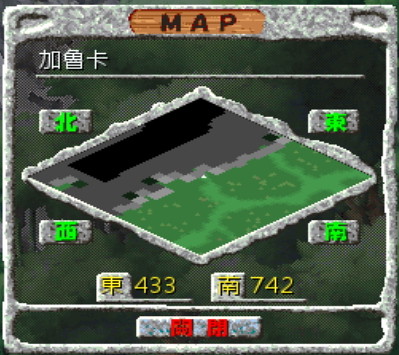The image showcases an in-game map interface from a video game, distinctively designed with retro pixelated graphics. The map is elegantly framed within a structure that resembles a worn metal casing, complete with screws at each corner, enhancing the nostalgic, old-school aesthetic. At the top of the frame, the word "Map" is prominently featured, accompanied by Japanese characters, adding a unique cultural touch. The map itself is rendered in an isometric perspective, offering a 3D representation of the game's terrain. The terrain is depicted in various shades of green, suggesting different elevation levels and topographical features. Below the map, numbers labeled in Chinese, "433" and "742," are displayed, likely serving as coordinates to assist players in navigating and locating their position within the game world.